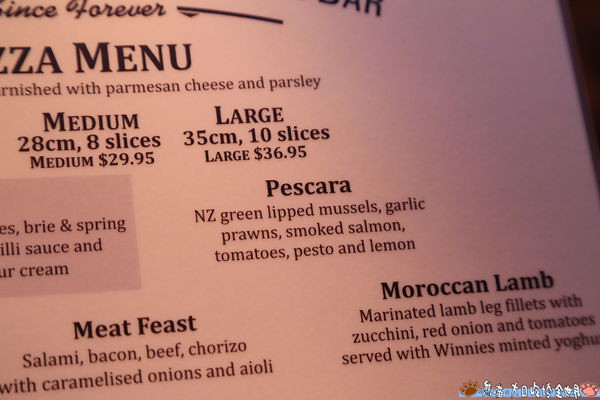This horizontally aligned rectangular image showcases a close-up of a restaurant menu with a distinct pinkish-purple hue, likely with a plastic coating. The upper left corner of the menu, with a plastic rim visible along the right edge, displays the partially obscured title "ZA menu." The visible text reveals dishes garnished with parmesan cheese and parsley. Bold black text further highlights options such as "Medium" and "Large," specifying sizes and prices—28 centimeters with 8 slices for $29.95 and 35 centimeters with 10 slices for $36.95 respectively. Additionally, detailed food descriptions include items like "Pescara" featuring NZ green-lipped mussels, garlic prawns, smoked salmon, tomatoes, pesto, and lemon. Beneath these, other options are listed in bold: "Meat Feast" with salami, bacon, beef, chorizo, caramelized onions, and aioli, and "Moroccan Lamb" detailing marinated lamb leg fillets with zucchini, red onion, tomatoes, served with Winnie's minted yogurt. The menu, captured indoors and filling the entire photo, features text in black, white, and an off-red color.